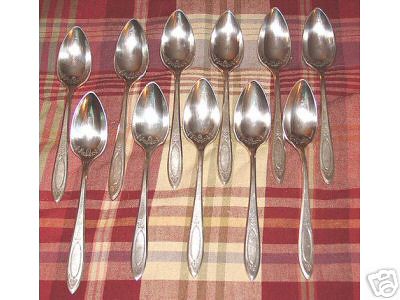The square image features a meticulously arranged set of 11 highly polished silver spoons reflecting the light, enhancing their lustrous appearance. They are laid out on a red and white plaid cloth, often described as gingham. The spoons, which may be teaspoons or fruit spoons due to their more pointed bowls compared to regular soup spoons, are placed in two rows. The top row consists of six spoons, and the bottom row holds five spoons. They are positioned in a zigzag formation, with the spoons in the bottom row nestled between the handles of the top row spoons, without overlapping. The handles of the spoons display an intricate filigree design, adding a touch of vintage elegance to the overall composition.